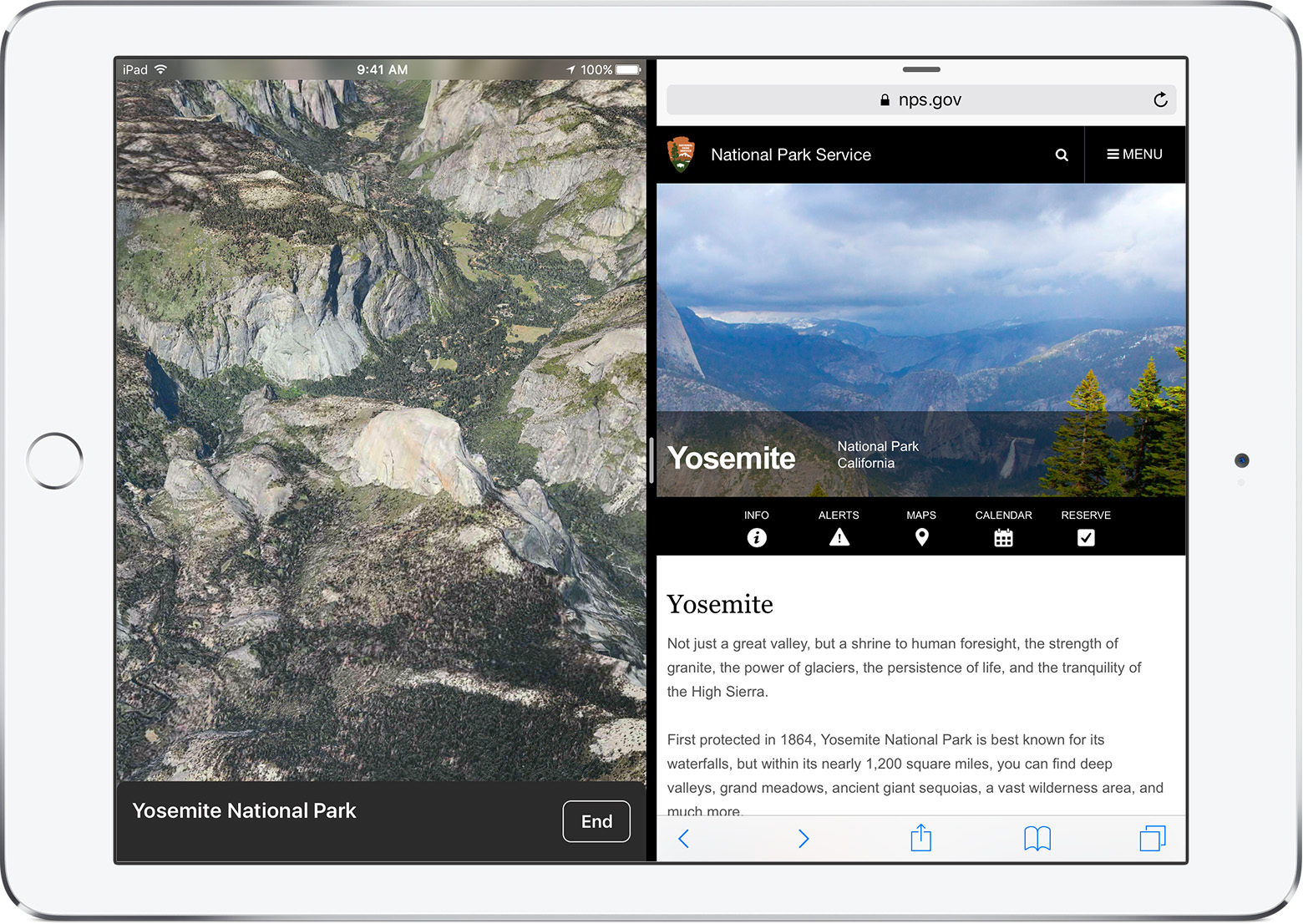This is a detailed screen capture of a website displayed on a horizontally oriented, Apple-style tablet. The tablet is white with a silver edge framing its design, and it features a silver circular button on the left-hand side, indicative of older iPad models.

The screen capture showcases the homepage of the Yosemite National Park section from the National Park Service's (nps.gov) website. Positioned prominently on the left side of the screen is a stunning photograph of Yosemite National Park from an aerial perspective, highlighting majestic mountains.

Directly beneath the photograph, a black bar reads "Yosemite National Park" and includes a button labeled "End."

On the right side of the screen, the National Park Service website header features the URL "nps.gov." Below this, a black navigation bar displays the National Park Service logo on the left, along with a search icon (magnifying glass) and a menu option.

Below the navigation bar and full-width across the display, another captivating scene of Yosemite's mountainous landscape is featured, adding visual depth to the webpage. Underneath this image, text reads "Yosemite National Park, California," accompanied by scenic pine trees in the foreground.

Following this, there are options for "Info," "Alerts," "Maps," "Calendar," and "Reserve."

An informative paragraph provides more context: "Not just a great valley, but a shrine to human foresight, the strength of granite, and the power of glaciers, the presence of life, and the tranquility of the high Sierra. First protected in 1864, Yosemite National Park is best known for its waterfalls, but within its nearly 1,200 square miles, you can find deep valleys, grand meadows, ancient giant sequoias, and a vast wilderness area - and much more."

At the bottom of the screen, there are navigation icons including back arrow, forward arrow, page up, save, and copy functionalities.